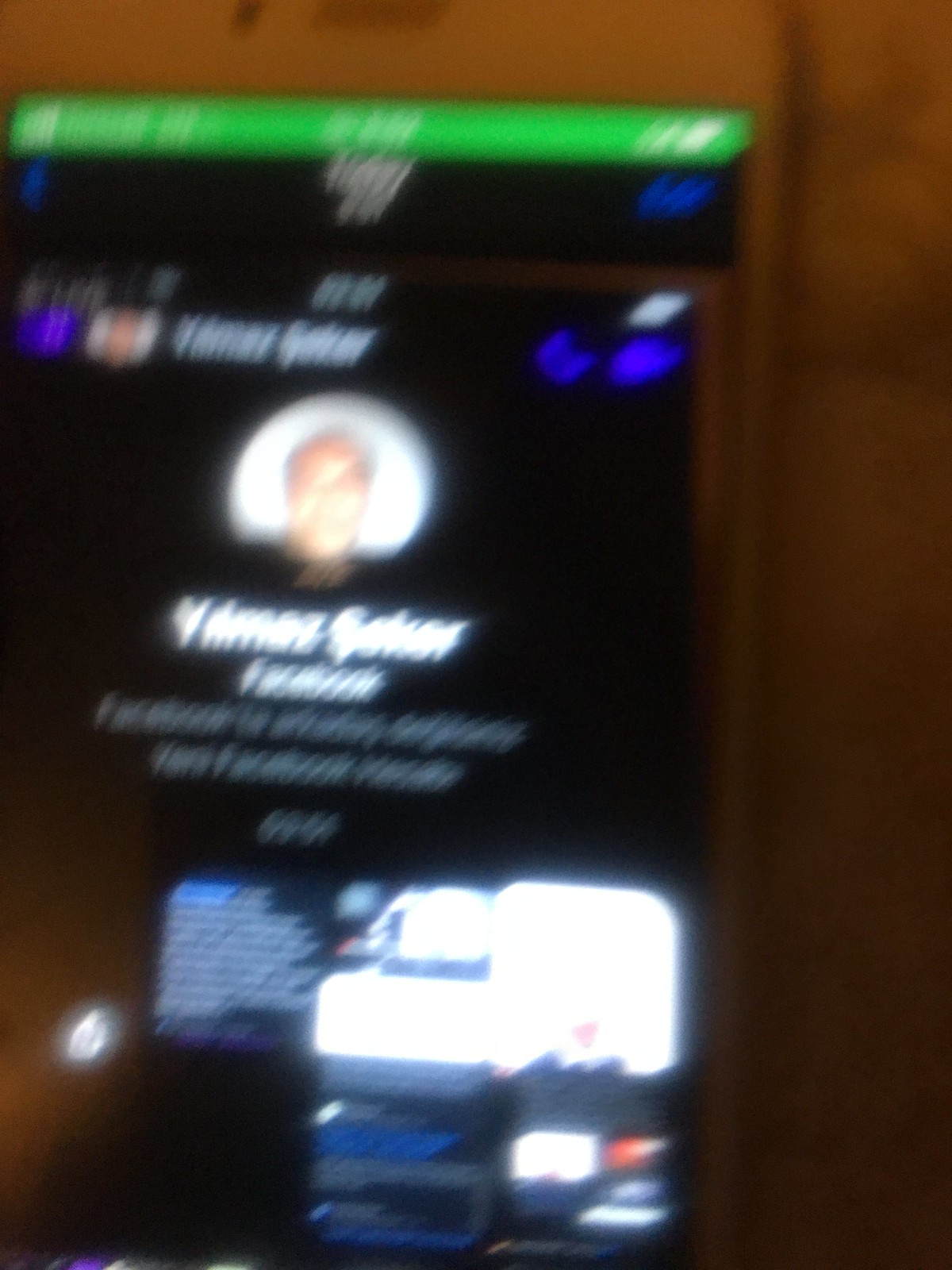A blurry photograph captures a cell phone screen, likely taken while the device was in motion. The screen shows a social media chat, indicated by the black background and layout typical of messaging apps. At the top of the chat, a partially legible name appears, possibly "Tammer" or "Tammy." Accompanying the name is the person's profile icon, depicting an individual with short red hair within a white circular frame. The individual seems to be wearing a dark sports coat over a yellow shirt. Below the name, the word "Facebook" is clearly visible in white text. The lower portion of the screen displays fragments of recent chat logs. The overall blurriness of the image obscures finer details, suggesting the photo was taken hastily or with an unsteady hand.